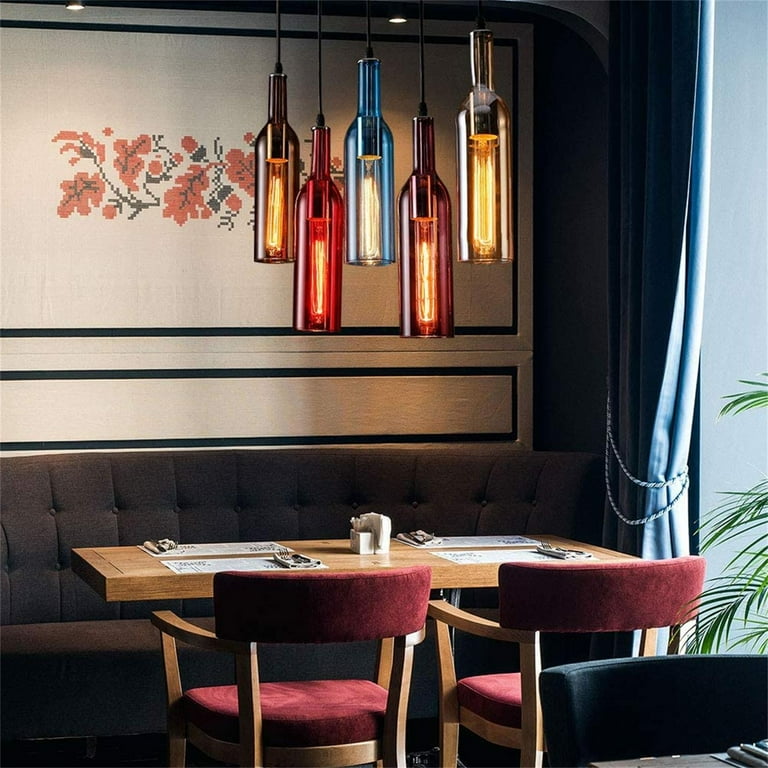The image depicts the interior of a cozy restaurant, featuring a wooden booth setup. At the center of the scene is a brown wooden table with four paper placemats and accompanying silverware neatly arranged. Each place setting includes a white napkin, with additional napkins and a sugar packet holder positioned in the middle. On the table, there are also salt and pepper shakers.

On the near side of the table are two wooden chairs with red velvet cushions on their seats and backs. Opposite the chairs is a dark gray or brown couch, offering comfortable bench seating. Above the table hangs a unique chandelier made of large glass bottle fixtures in various colors: orange, red, blue, burgundy, and yellow, each housing long filament-style bulbs.

The background reveals a wall adorned with red and green floral designs. Additionally, a small plant is visible peeking through a nearby window, adding a touch of natural charm to the restaurant's warm and inviting ambiance.